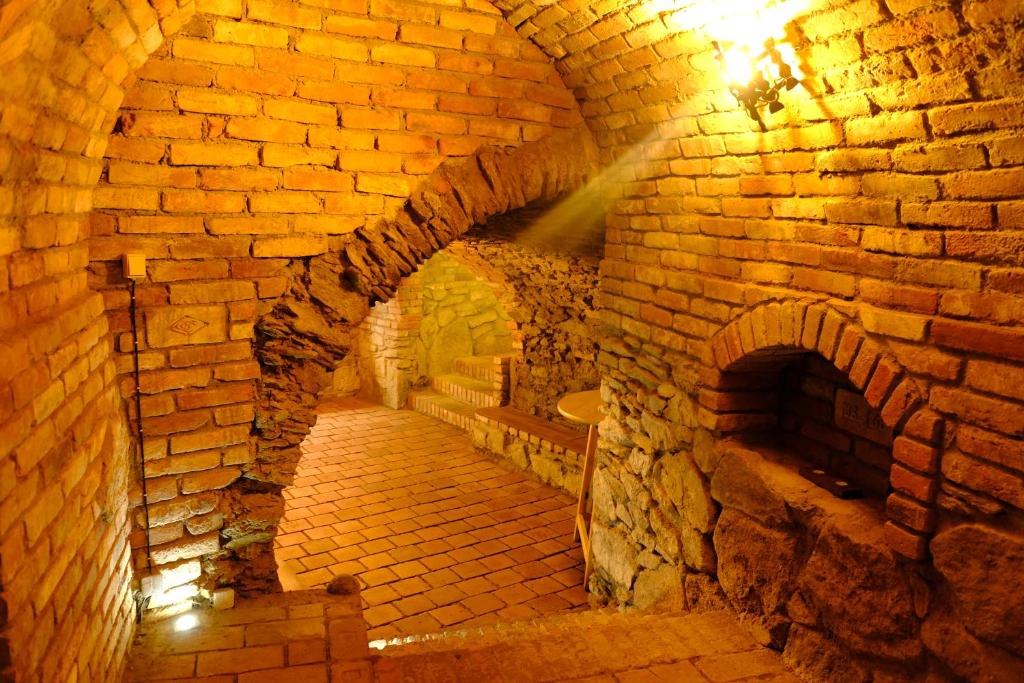The image depicts an underground brick passageway, intricately constructed with an arched ceiling, and fully lined with brown and yellowish-brown bricks. On the right side of the passage, an arched brick oven is seamlessly built into the wall, distinguished by its rounded border. There is also a small brick bench or stool on the left side, providing a place to sit. The floor is similarly made of bricks, and a light source emanates from the upper right corner, casting a warm yellow glow over the scene. In the center of the photo, the passageway features a small step down leading to another arched doorway, partially walled off with a semicircular cutout that aligns with the overarching shape of the space. This cutout allows for passage through the structure. The scene hints at further exploration with hints of stairs and additional archways extending beyond what is visible in the image.